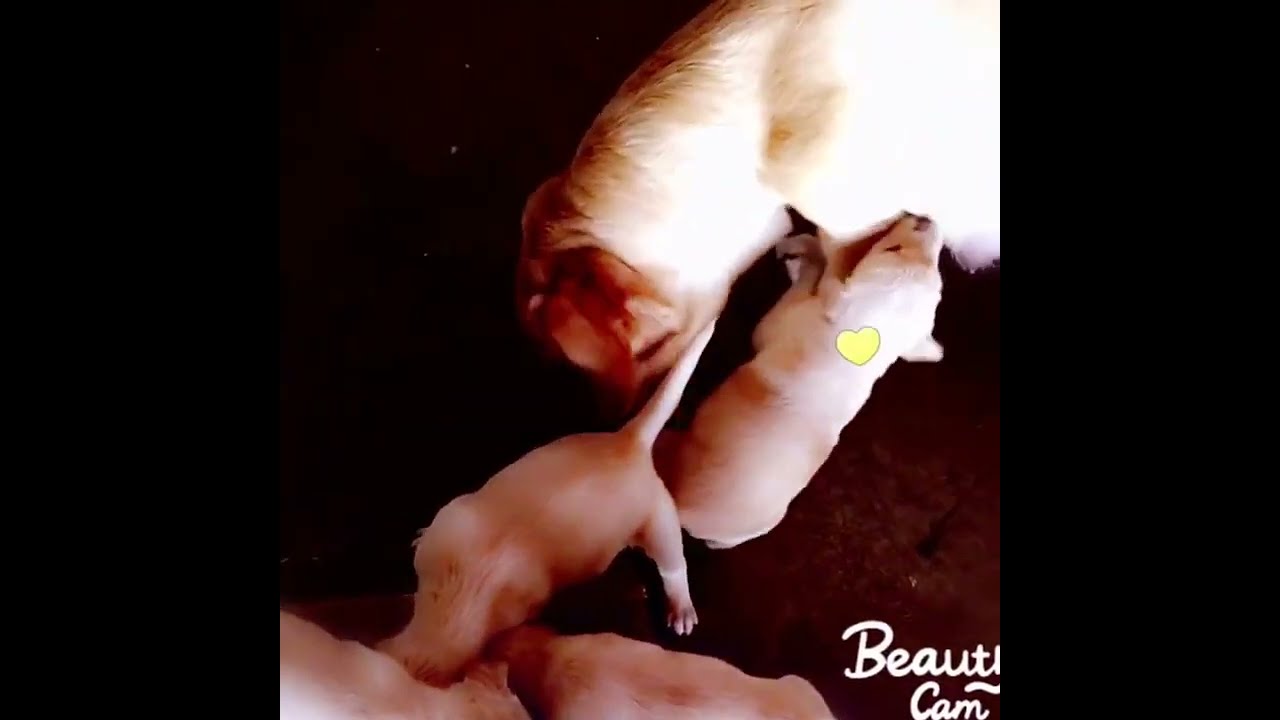The image depicts a scene with a mother golden retriever and her three light-colored puppies. The puppies are positioned at the bottom of the image, with one puppy appearing to nurse from the mother dog, whose head is tilted downward and towards the center of the photograph. The mother's tail is pointed upwards while one of the puppies is located in front of her, and another to the middle right. A small yellow heart graphic is placed above the nursing puppy's neck, and the overall background is dark brown. On the lower right corner, the partially cropped text "Beauty Cam" in white cursive lettering is visible. There are vertical borders on the left and right sides of the image, enhancing the focus on the dogs.